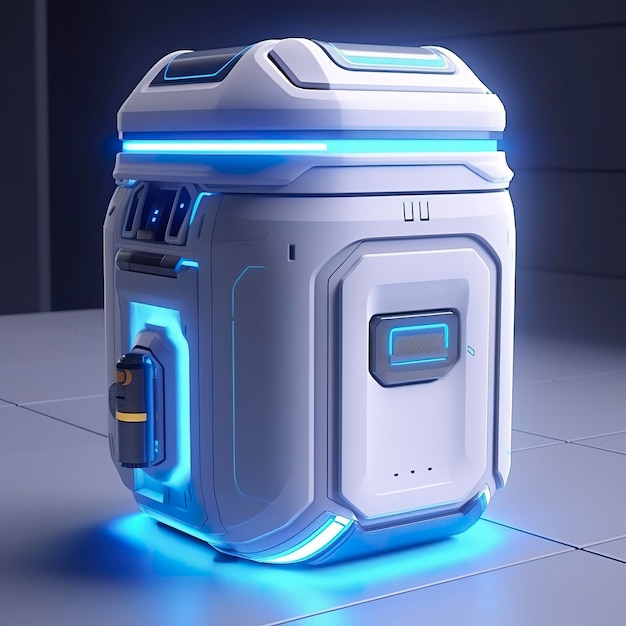The image depicts a highly detailed, AI-generated 3D scene featuring a futuristic, robotic-looking device. The rectangular, canister-like structure is primarily white with a smooth, plastic-like surface and is embellished with various lights and buttons. A striking blue neon glow emanates from rings bordering both the top and bottom edges of the device, casting a reflective bluish light onto the white, tiled floor below. This glow highlights a yellow-striped gray canister integrated into the machine. The background showcases a minimalist gray wall, adding to the digital, high-tech ambiance reminiscent of environments from video games like Overwatch or Portal.